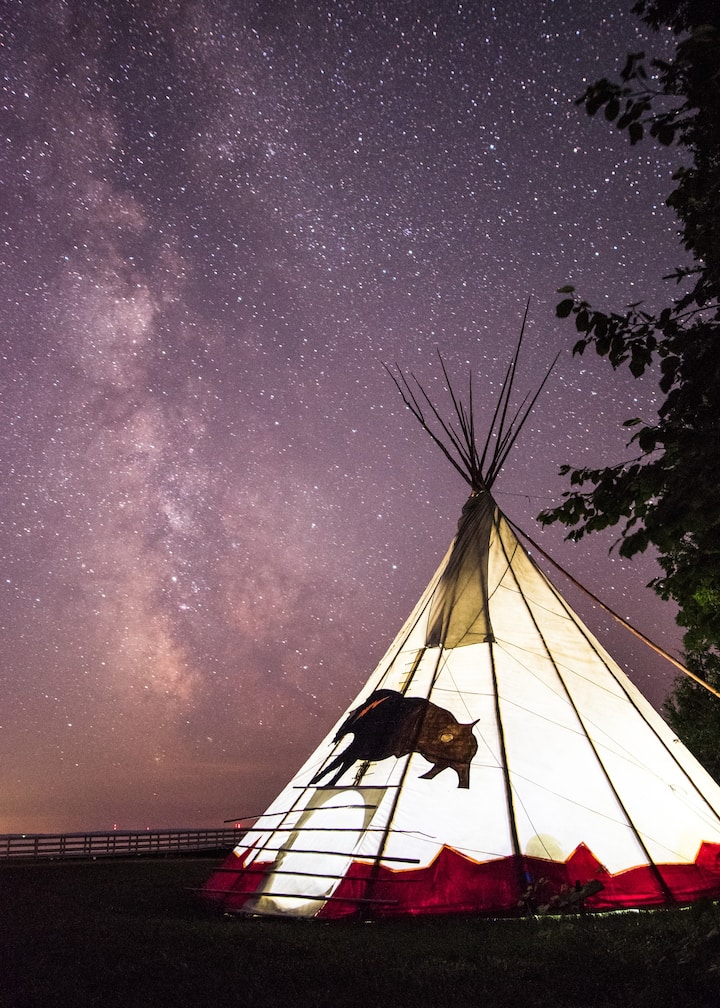Under a night sky glimmering with countless stars, a white teepee with a red base stands illuminated, casting a serene glow against the dark backdrop. A faint image of a buffalo or bison adorns its side, and near its lower section, a small square doorway is visible. The teepee is supported by multiple poles converging at the top. To the right of the image, tall trees stretch upwards, their silhouettes reaching to the top. On the left, a distant fence suggests the presence of water beyond, while dark, grassy terrain covers the ground. The overall ambiance of the scene is tranquil, accentuated by the soft, ethereal light of the teepee under the majestic starlit sky.